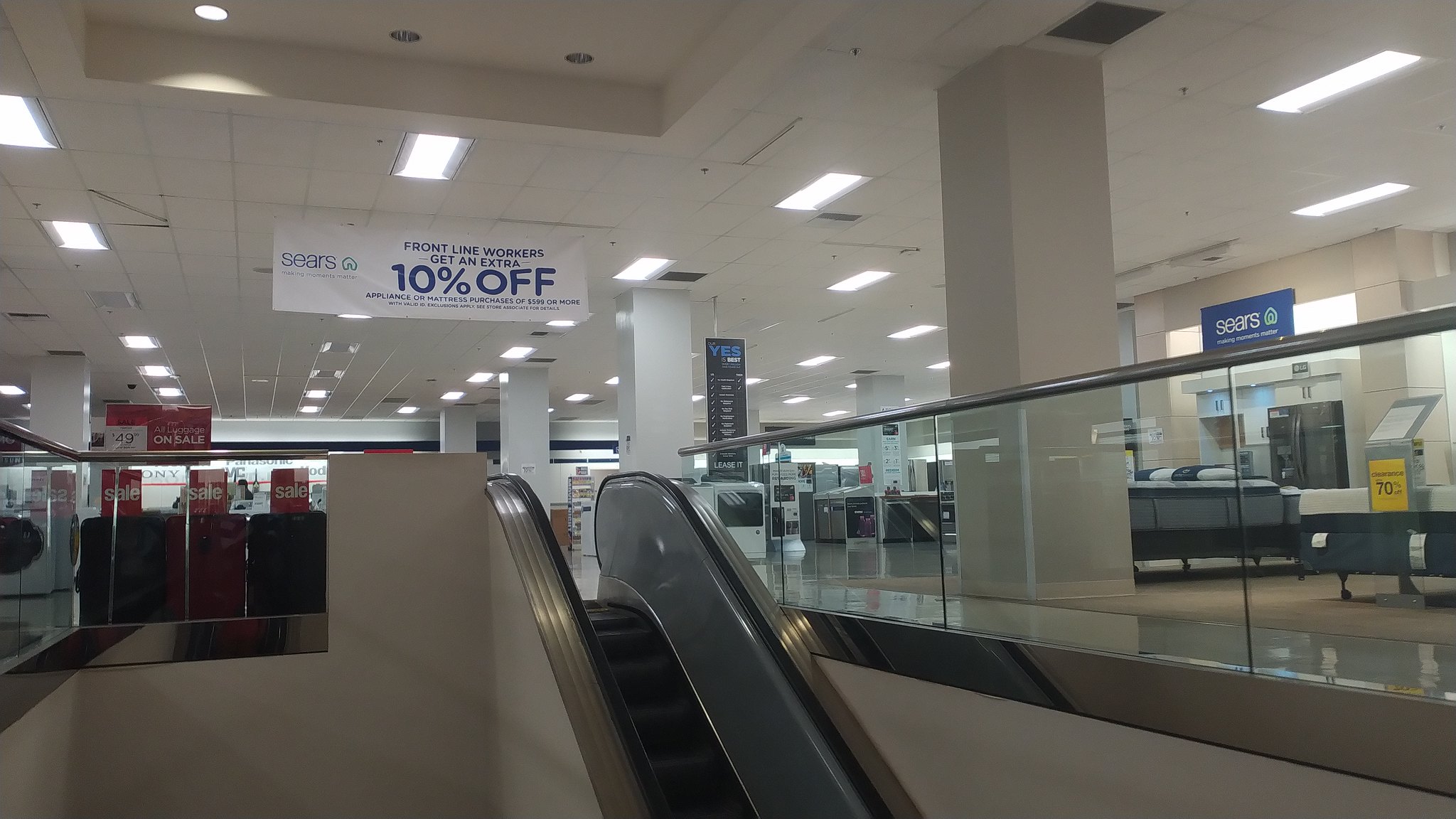The photograph shows the interior of a Sears store, capturing a detailed view of the top floor. Dominating the foreground is the top of an escalator, with its sleek silver handrails glinting under the store's lighting. Surrounding the escalator's opening are half-walls made of clear glass, allowing an unobstructed view of the store’s merchandise. Along the top edge of these glass walls runs a continuous silver handrail.

Hanging prominently above the escalator is signage announcing a 10% discount for frontline workers, likely a measure implemented during the COVID-19 pandemic. The store's layout reveals various sections, including a furniture area. A bright yellow sign draws attention with a "70% off" discount. Visible pieces of furniture include a bed and a dresser, though other background images are less distinct.

The store's architecture includes supporting columns and a flat ceiling fitted with recessed lighting panels. Additional sales signs are visible on the left side of the image, though the specifics of those promotions remain unclear. Overall, the image encapsulates the commercial atmosphere of a retail space keen on attracting customers with significant discounts.